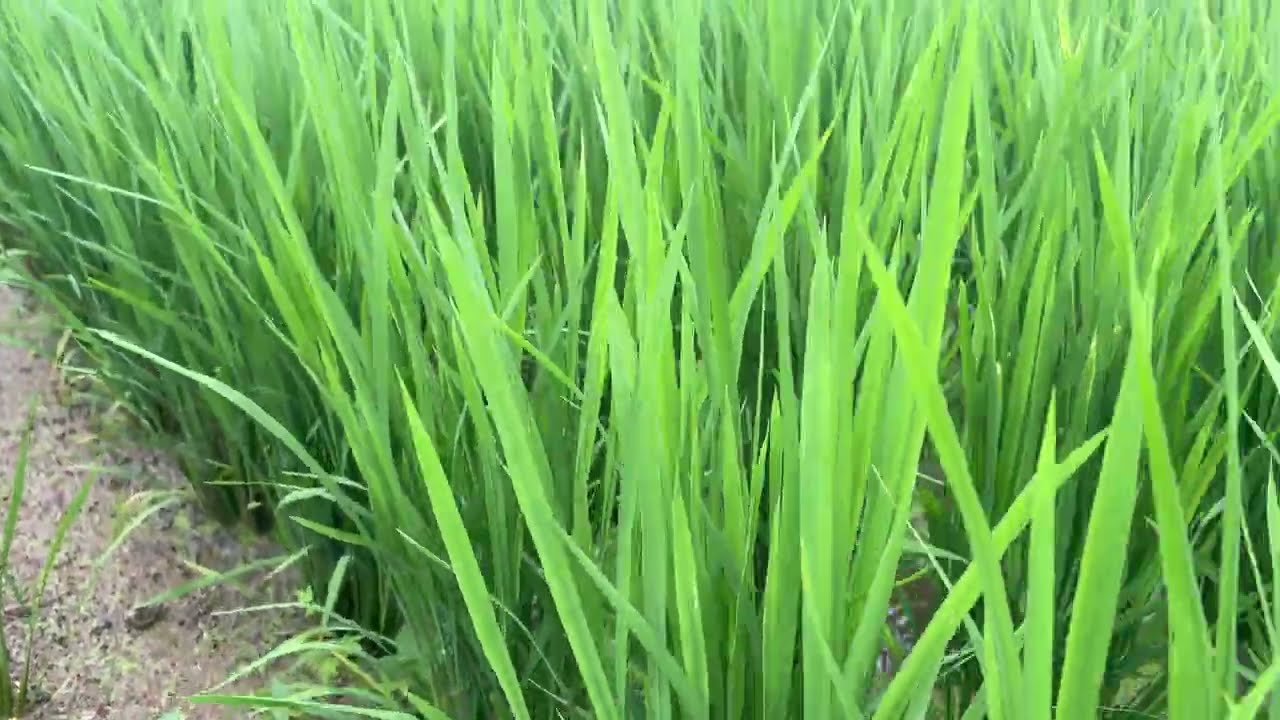This is a striking macro photograph capturing blades of chartreuse and varying shades of green grass, growing tall and upright from the soil. The blades of grass are approximately 10 inches in height and dominate almost the entire image, with a distinct patch of sandy, wet earth visible in the bottom left corner. In this section, you can spot a few worms amidst the loose grayish-brown sediment, speckled with small pebbles and fragments. The grass appears dense and lush, arranged in clumps that give the impression of rows. The interplay of light and shadow highlights the different shades of green, with some blades appearing almost yellowish chartreuse while others are darker green. The sunlight creates a contrast, illuminating the outer leaves while the inner parts remain in shadow, adding depth and texture to the scene. No people, vehicles, or buildings are present in the image, allowing the focus to remain solely on the natural beauty of the grass.